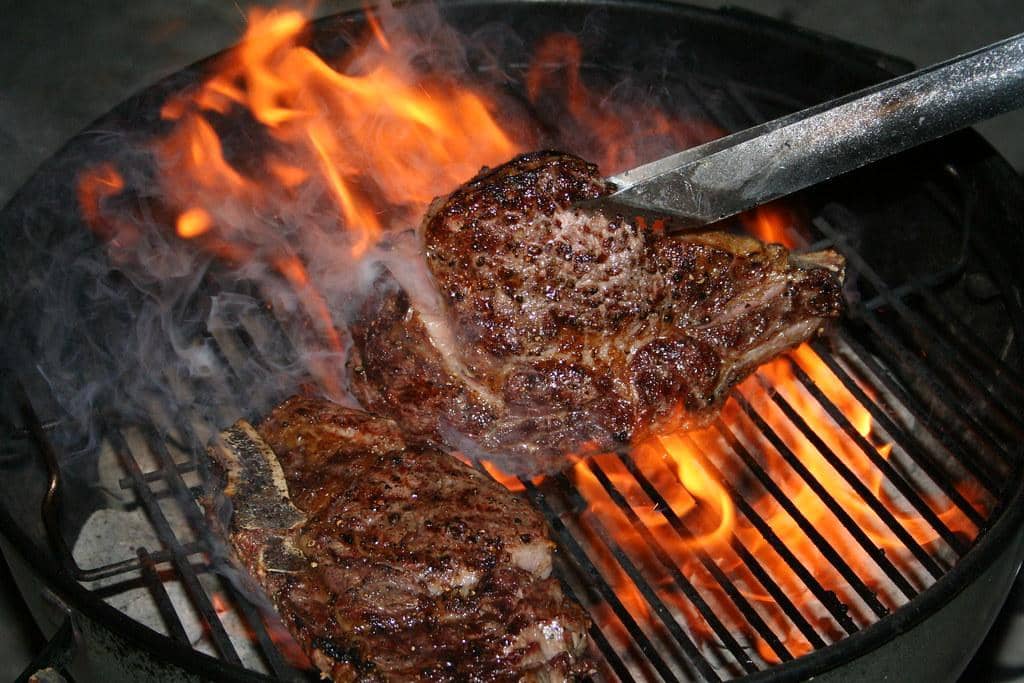A close-up image of a circular charcoal grill features two pieces of meat, likely pork chops, grilling over an open flame. The grill's grated surface, marked by numerous crisscrossing black slats, is glowing with an intense yellowish-orange fire that sends up plumes of white, ashy smoke. One piece of meat is held by a pair of metal tongs from the right side of the image, appearing either to be placed onto or flipped on the grill. The meat, possibly pork chops given its color and shape, displays a variety of hues from tender light brown and tan on the inside to charred dark brown and blackened spots on the outside. The scene is intense with flames licking up around the edges of the meat, creating an atmosphere of high heat cooking. The background of the image is a dark gray, seamlessly blending into the upper left corner, adding to the focus on the grilling action.